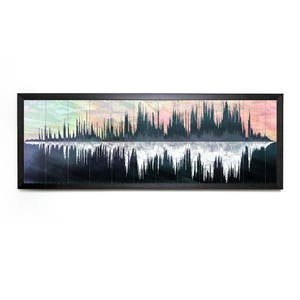The image is of a small, tightly compressed piece of art with a detailed scene. It features a long horizontal rectangle framing jagged black lines that rise up and down like a cardiogram. These lines are depicted in two sections: the top section showcases a colorful gradient sky transitioning from greens on the left side to oranges, purples, pinks, and dark pinks on the right side, creating a vivid sunset effect. In contrast, the bottom section mirrors these jagged lines but in black and white, resembling the reflection of the top scene on water. The entire image is encased in a medium to dark brown frame, which complements the artwork's dynamic range of colors and textures. Despite its small size, almost like a thumbnail, the piece captures a striking visual of a sunlit sky with jagged black forms that may evoke the imagery of a skyline or trees, and their white reflections on a dark surface below.